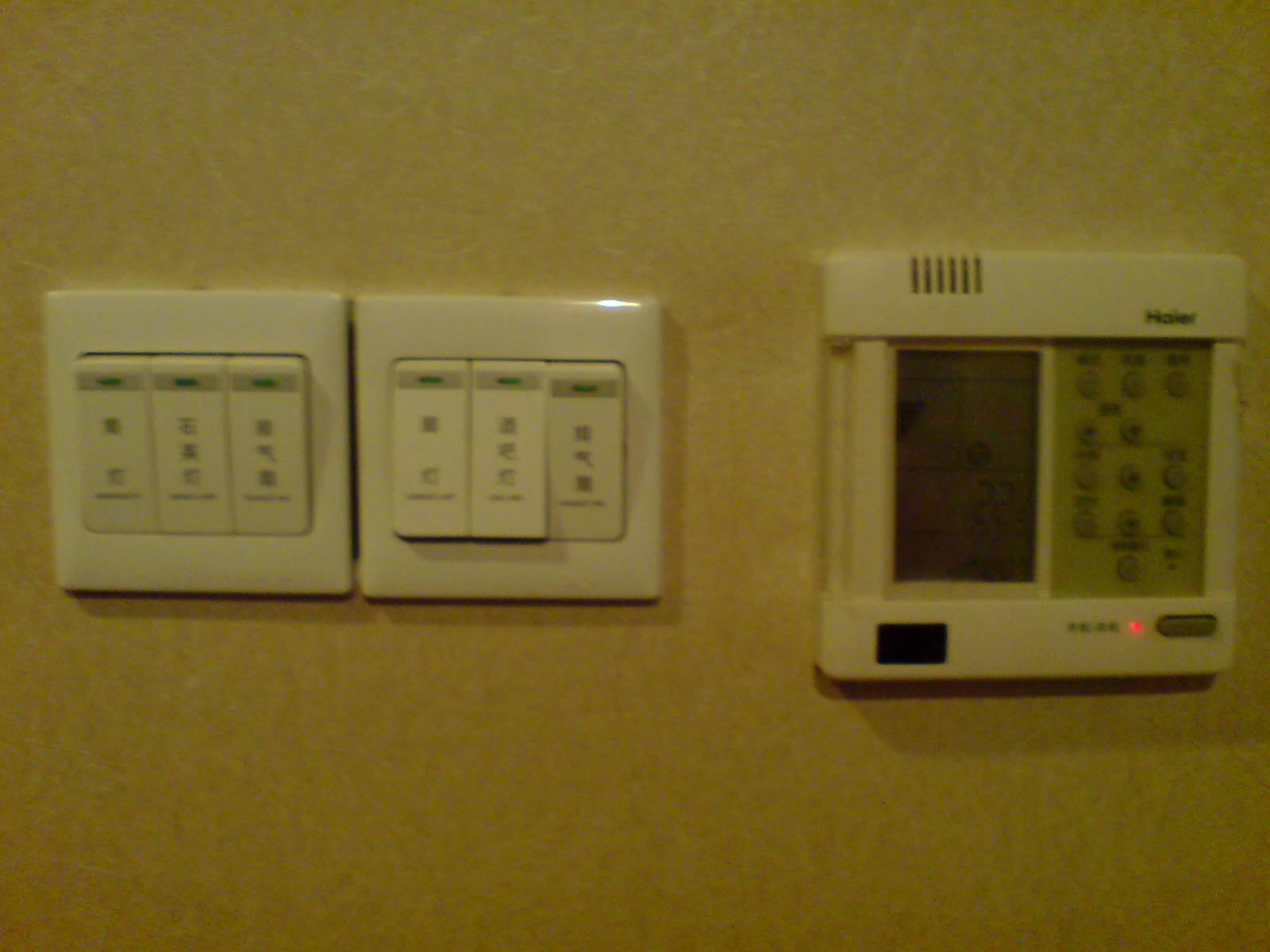The image is a color photograph, albeit significantly out of focus and blurry. The primary focus appears to be on a group of heating and air temperature controls mounted on a wall. The wall itself seems to be textured and painted in a beige or tan color.

On the left side, there are two identical ivory-colored square plastic switch plate covers. Each cover houses three vertical rectangular buttons inscribed with Chinese characters. Above each button is a shaded area featuring a sideways rectangle, which appears to be an indicator that lights up, likely with a green lens. On the second set of buttons, the rightmost button is pressed in while the others remain in their default positions.

A few inches to the right of the switch plates is a thicker and sturdier control unit bearing the brand name "Haier," known for producing air conditioners. This unit has small vents at the top, which could either be for ventilation, wiring for a thermostat, or even a speaker. The control panel features a large digital screen displaying the number "22," with other, unreadable information also present. Below the screen, there is a panel of round buttons with labels that are too blurry to decipher.

At the bottom left of this control panel, there is a dark rectangle, its purpose unclear—it could be a label, a light indicator, or a rocker switch. Additionally, there is a small red lens that is glowing, suggesting it is an active indicator light.